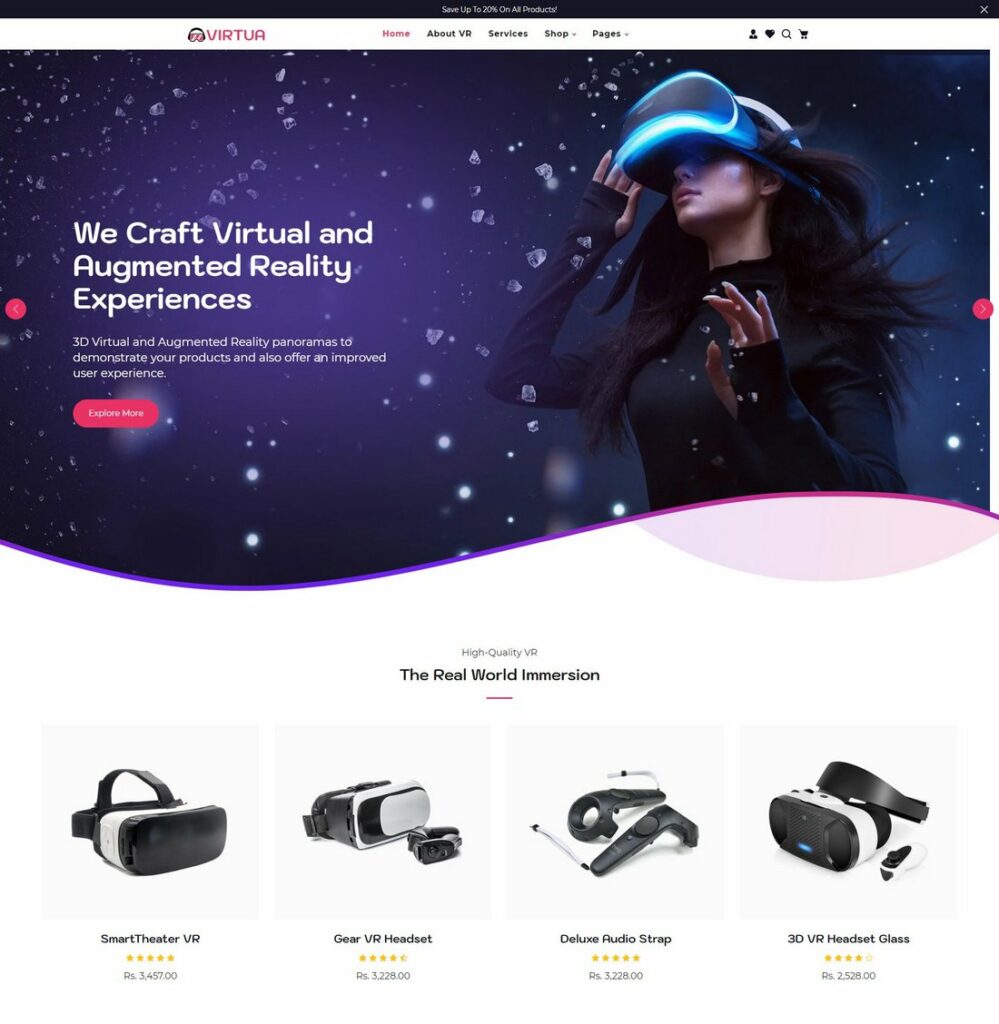This advertisement features a banner at the top, encased in a blue rectangular box adorned with a sparkling bubble design. Prominent white lettering announces: "Recraft Virtual and Augmented Reality Experiences: 3D Virtual and Augmented Reality Panoramas to Demonstrate Your Products and Offer an Improved User Experience." Just beneath, a link invites viewers to "Explore More."

To the right, a striking image of a model captures attention. The model's face, incredibly smooth as if computer-generated, suggests an otherworldly aesthetic. She has long, dark hair dramatically flowing, wearing thick 3D glasses illuminated by a blue light. With one hand, she touches the glasses while clad in a long-sleeved black turtleneck, exuding a neutral expression.

Below this, a lineup of additional products is showcased, emphasizing "High Quality Virtual Device Experience (VDE)" for real-world immersion. Featured items include:

- **Smart Theater VR:** Priced at $3,457.00
- **Gear VR Headset:** Priced at $3,228.00
- **Deluxe Audio Strap:** Priced at $3,228.00
- **3D VR Headset Glass:** Priced at $2,528.00

Each product promises to elevate the virtual reality experience, underscoring the advertisement’s commitment to cutting-edge technology and immersive interactions.